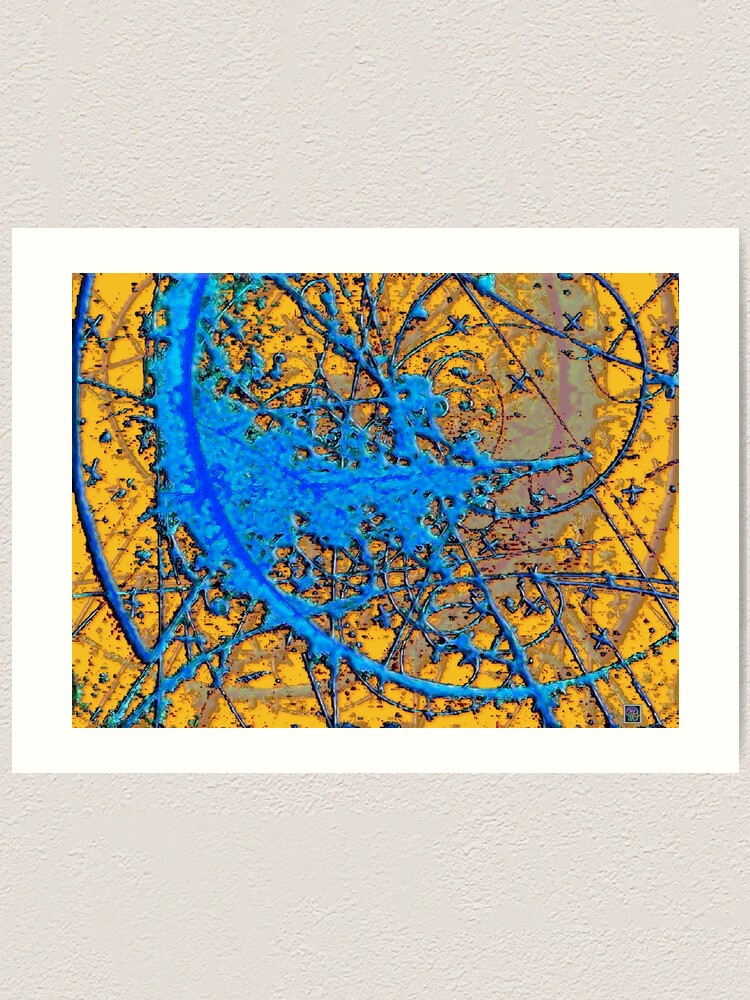The image is an abstract, modern painting mounted on a white mat and set against an off-white or light gray textured wall. The painting features a mustard yellow background with vibrant blue paint splatters, drizzles, and circular patterns dominating the foreground. There are also some dark black or brownish lines and shapes intermixed with the blue swirls, giving the piece a layered appearance. The overall design is reminiscent of Jackson Pollock’s style, with chaotic yet aesthetically pleasing splashes and strokes. The entire artwork, set within a white frame, sits on a beige rectangular background, adding to its striking presence. The detailed texture and interplay of colors create a dynamic, visually engaging piece that catches the eye.